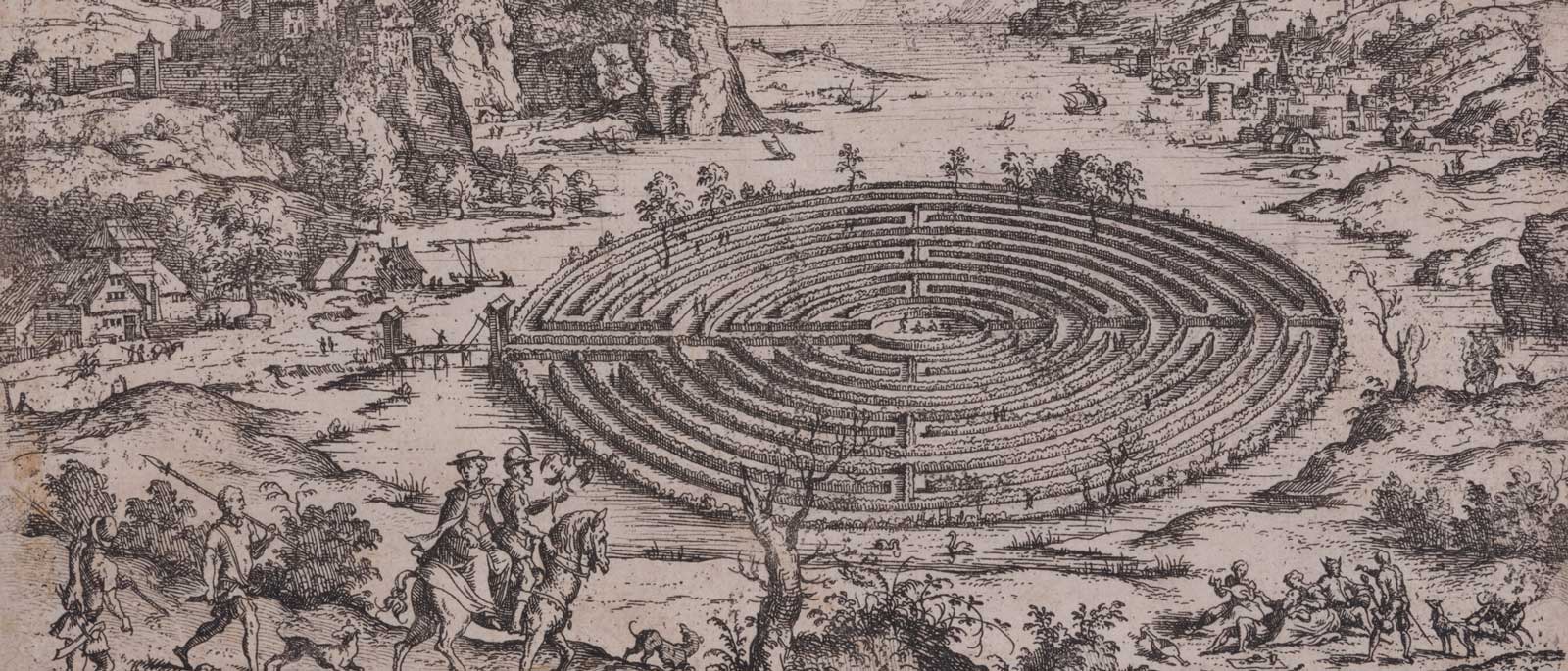This intricate black and white drawing captures a historically evocative scene brimming with activity and detail. At the heart of the illustration is a large, circular maze, resembling a labyrinth, with meticulously trimmed hedges or trees forming the intricate paths. This maze is set on an island, encircled by a water moat, necessitating the crossing of a bridge to enter. The bridge connects to a tract of land on the left, featuring a multi-story house with a horse-drawn carriage in front.

The bottom left corner of the drawing showcases a dynamic array of figures, including a man and woman on horseback, the man holding a falcon. Nearby, a figure with a sword over his shoulder, another identified as an Indian with a long headdress, and several dogs add to the scene's bustling nature. In the maze itself, people walk along its paths, engaged in various activities. 

To the right, there's a group of women playing instruments, accompanied by a dog and possibly a man. Birds are scattered throughout, adding life to the scene. In the far distance, grandiose medieval-like castles and fortresses atop rocky hills overlook the entire setting, with mountainous terrain offering a dramatic backdrop. The image reflects a tableau from a bygone era, possibly medieval or colonial, bustling with life and rich in detail, inviting viewers to ponder its historical and geographical context.